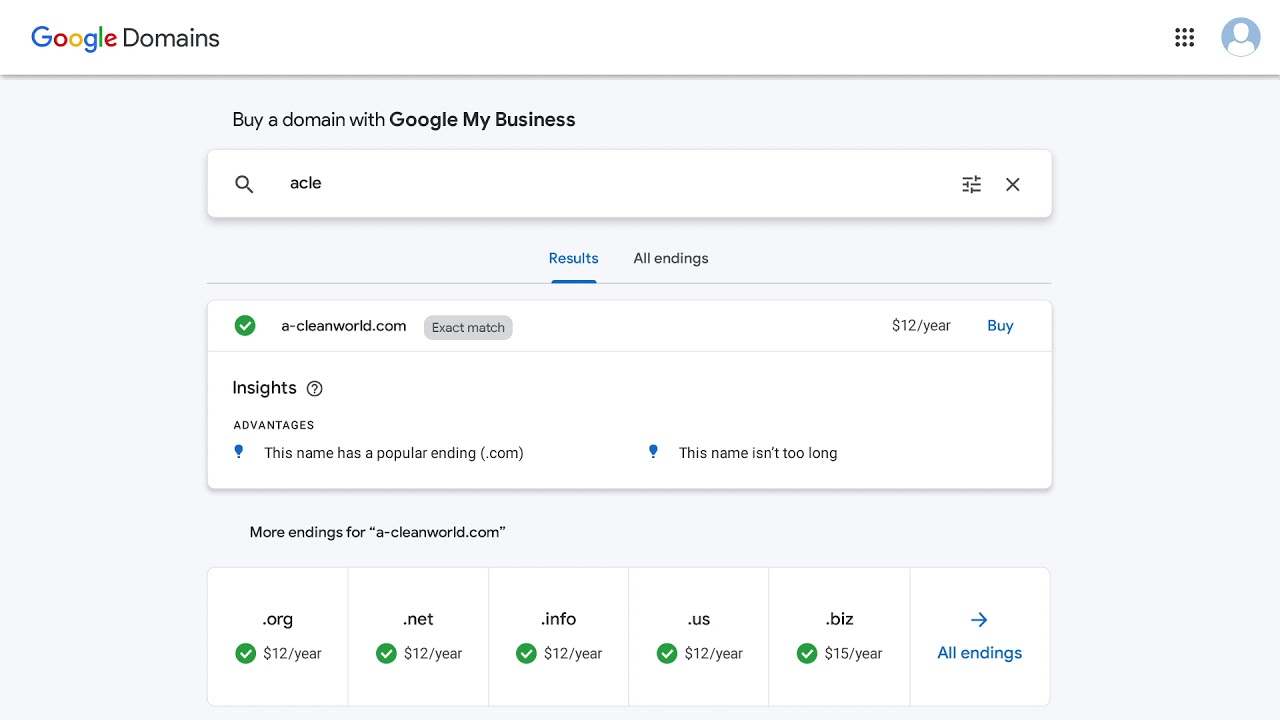This image is a screenshot of a Google Domains page. The overall background is pale gray, while the main content is displayed in white boxes. 

At the top of the image, the header is white. On the top left corner, "Google Domains" is written with "Google" displayed in its signature colors: blue, red, yellow, blue, green, and red. In the top right corner, there is a profile icon, represented by a circle containing a stylized image of a person, and to its left, there is a grid icon made up of nine dots forming a square, which serves as the menu button. Beneath this header is a thick gray line separating it from the main page content.

The main section begins with the title "Buy a domain with Google My Business." Just below this title is a white text box accompanied by a magnifying glass icon on its left, indicating a search function. It appears that someone has entered text, likely "ACIE" or "ACLE," into this box. To the right of the text box, there are two icons: a settings option and an 'X' to close it.

Further down, there are two tabs: "Results" and "All Endings," with "Results" currently highlighted in blue. This section reveals that the exact match domain "acleanworld.com" is available for $12 per year and includes a "Buy" button running across the bar. Below this, an "Insights" section details the advantages of this domain name, mentioning it has a popular ".com" ending and is not too long.

Another heading, delineated against the gray background, reads "More endings for acleanworld.com." The following white box lists additional domain options, all priced per year: ".org" for $12, ".net" for $12, ".info" for $12, ".us" for $12, and ".biz" for $15. On the far right of this box is a right arrow labeled "All Endings" in blue, which can be clicked to view more domain extension options.